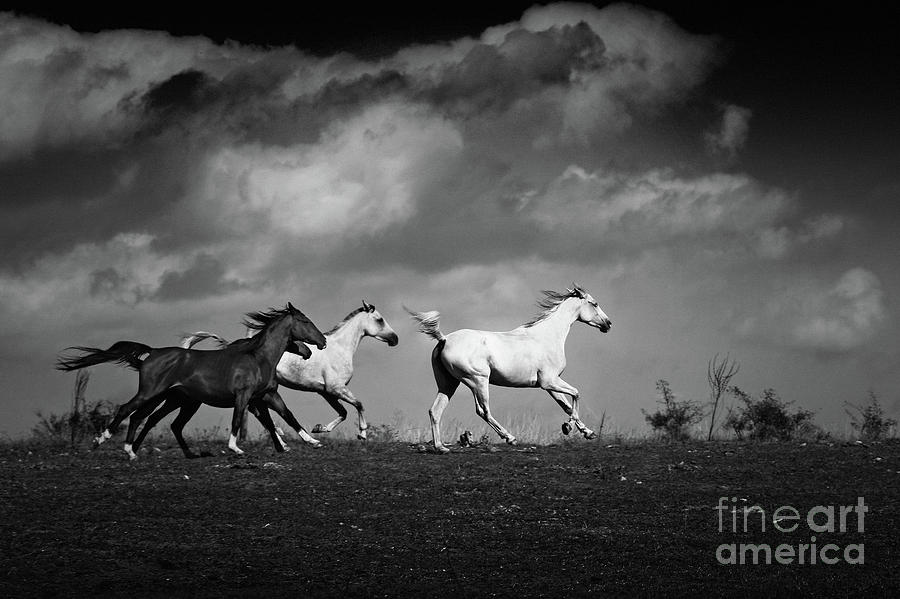This black-and-white photograph, reminiscent of fine wall art, captures an evocative scene of wild horses running through a dark, ominous field. The dramatic sky above is filled with brooding black and grey clouds, enhancing the tense atmosphere. The composition features two prominent white horses leading the charge, followed closely by two smaller, darker horses—likely black or brown—all in mid-stride, their manes and tails flowing in the wind. The ground they traverse is a stark, black dirt field dotted with patches of shrubs and bushes. The overall mood is one of movement and intensity against a backdrop of impending stormy weather. In the lower right-hand corner, the image is marked with "Fine Art America."